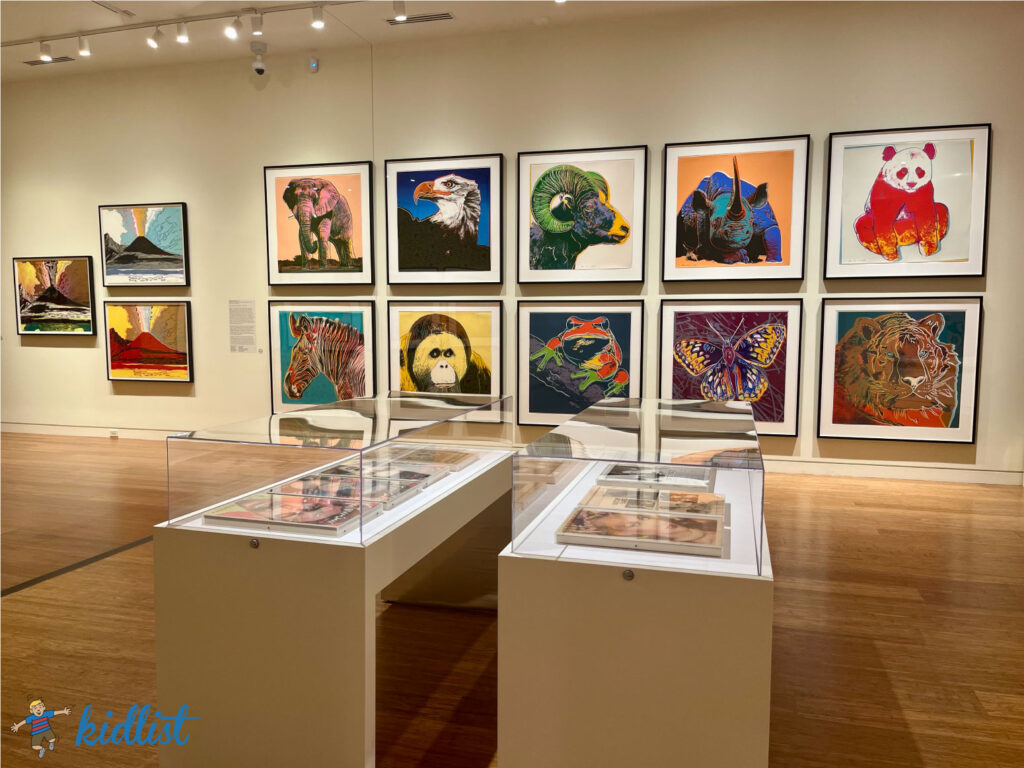The image depicts the interior of an art gallery with meticulously polished hardwood floors. Dominating the scene is a long wall adorned with a series of square frames, arranged in two horizontal rows, illuminated by track lighting from above. The frames display vividly colored images of various animals including a panda, zebra, rhino, butterfly, eagle, elephant, frog, monkey, tiger, and long-haired sheep, with themes ranging from wildlife to vibrant insects. Notably, three additional frames on the left side of the wall capture different eruptions of volcanoes, each rendered in distinct color schemes of red, black, and black with water. In the foreground, two display cases with white bases and plexiglass tops encase additional pictures laid out flat. At the bottom left corner of the picture, the text "Kid List" appears in blue cursive, accompanied by an emblem of a little boy with outstretched arms.